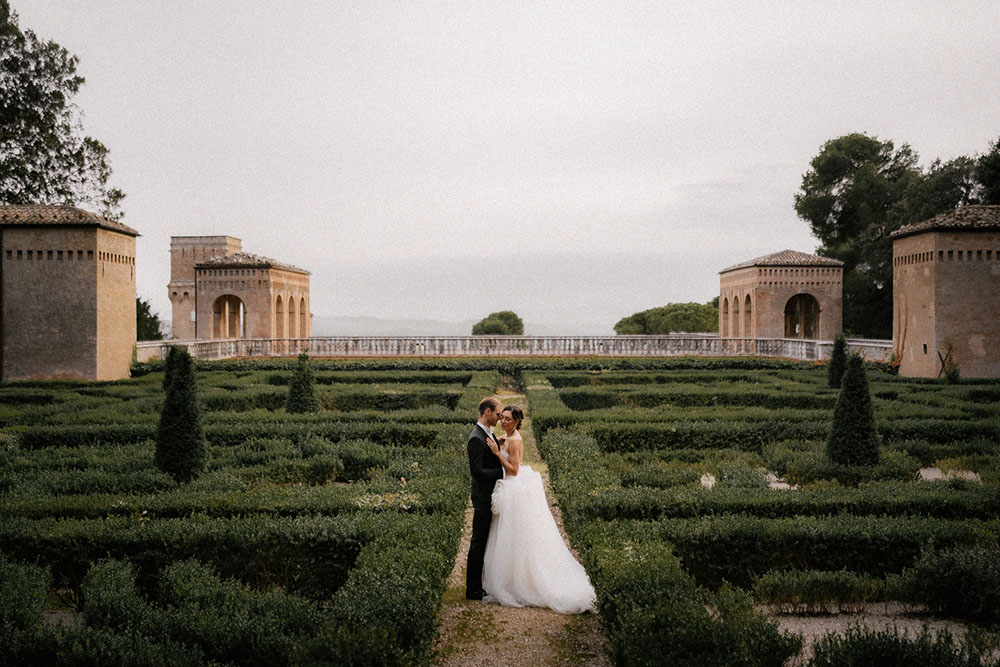In this detailed outdoor wedding photograph, the scene is set under a milky gray overcast sky, occupying the upper half of the image. The bride, in a white wedding dress with a puffy skirt, and the groom, in a black tuxedo, are standing closely on a gravel walkway in the center of a large, meticulously designed hedge garden. They hold each other lovingly, the bride's hands resting on the groom's chest while his arms wrap around her waist. The garden is an elaborate maze of knee-high, green, squared hedges with intricate designs within the squares. Four small trees stand within this maze, two on each side of the couple. In the background, tan stone buildings and other structures dot the landscape, framed by a fence that stretches across the middle distance, beyond which the serene overcast sky looms.